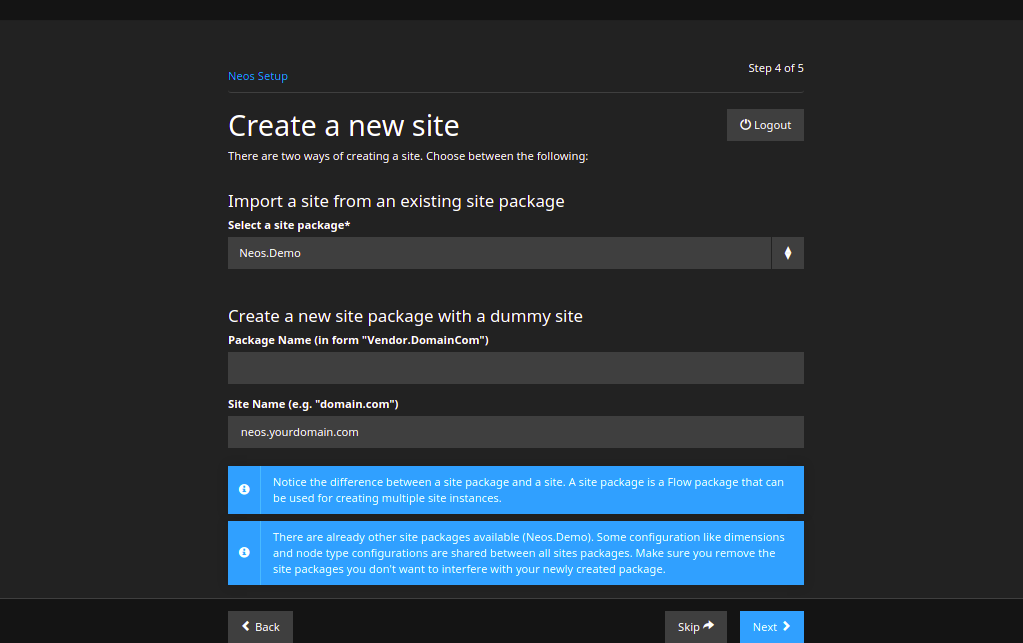The image is a screenshot of a configuration section of a website titled "Create a New Site," identified as Step 4 of 5. The section's header, "Neo's Setup," is prominently displayed on the left.

Below the header, the instructions explain the two methods available for creating a site:
1. "Import a Site from an Existing Site Package" with a selectable field that currently displays "Neo's.demo."
2. "Create a New Site Package with a Dummy Site," where users can input a package name, noted as "informvendor.domain.com." This field is currently empty.

Additionally, there is a field labeled "Site Name" with an example format "e.g., domain.com," which is currently filled with "neo's.yourdomain.com."

Two notices provide important information:
1. "Notice the difference between a site package and a site. A site package is a flow package that can be used for creating multiple site instances."
2. "There are already other site packages available."